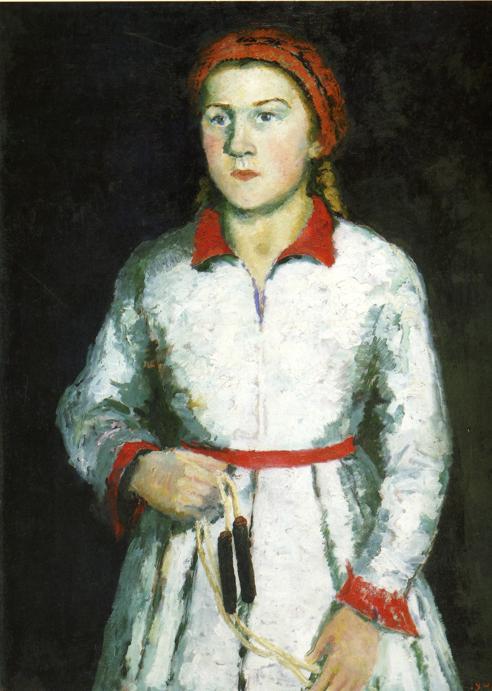This painting depicts a young girl, approximately 12 years old, against a dark, almost black background. She is adorned in an old-fashioned white dress featuring red trim details on the collar, belt, and cuffs. Her attire is complemented by a red and orange scarf or bonnet that partially covers her golden or light brown hair, with two ringlet curls cascading on each side. The girl's face is framed beautifully with her dark blue eyes and pouty lips, tinted red, and her cheeks holding a soft, flushed pink hue. She stands in a serene, relaxed manner, looking slightly to the left of the viewer with a stoic expression. In her hand, she holds an object resembling a jump rope with two handles at the end of a cream-colored rope. The painting captures the girl's subtle yet determined demeanor with a serene essence, accentuated through the less precise, yet evocative brushstrokes.